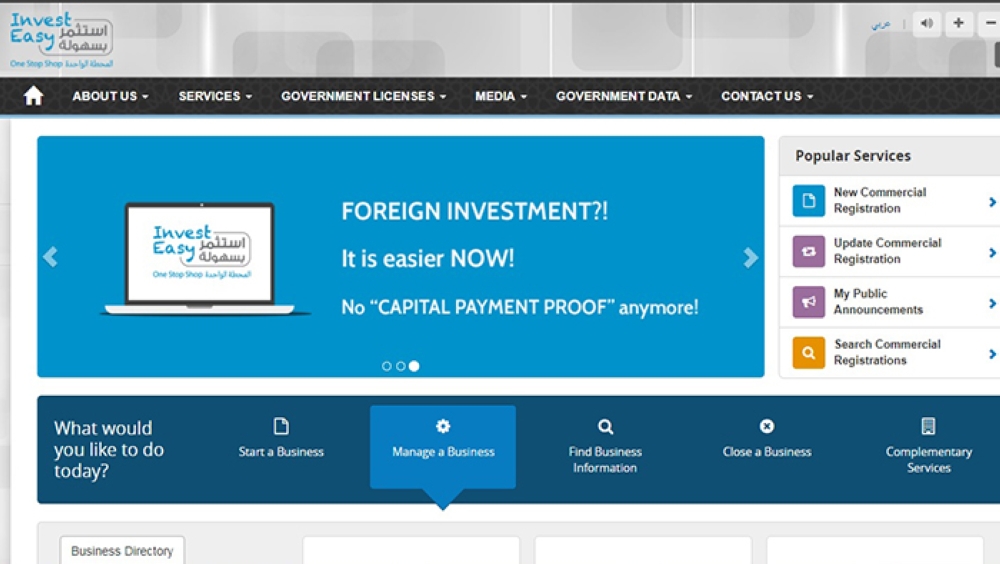This image is a detailed screenshot from a website featuring an intricate and well-organized layout. At the very top, the header is designed with a subtle gray pattern consisting of squares in varying shades and rounded corners. On the left side of the header, the company name "InvestEasy" is prominently displayed in a blue font, followed by its Arabic translation in a gray font.

Below the header, the main menu is presented against a black background, with the options highlighted in white font: About Us, Services, Government License, Media, Government Data, and Contact Us. Central to the layout is a distinct blue background section, with bold white text that reads "Foreign Investment‽ It is easier now! No capital payment proof anymore."

On the left side of this section, there is an illustration of a laptop screen, displaying the same InvestEasy logo in blue (English) and gray (Arabic). On the right side of the screen, the sidebar is labeled "Popular Services" and lists four specific offerings: New Commercial Registration, Update Commercial Registration, My Public Announcements, and Service Commercial Registrations. 

Beneath this, a darker blue border hosts a white-font question: "What would you like to do today?" Below the question, several options are available, including Start a business, Manage a business, Find business information, and Choose a business. Additionally, on the right side of the screen, there is a section titled "Complementary Services."